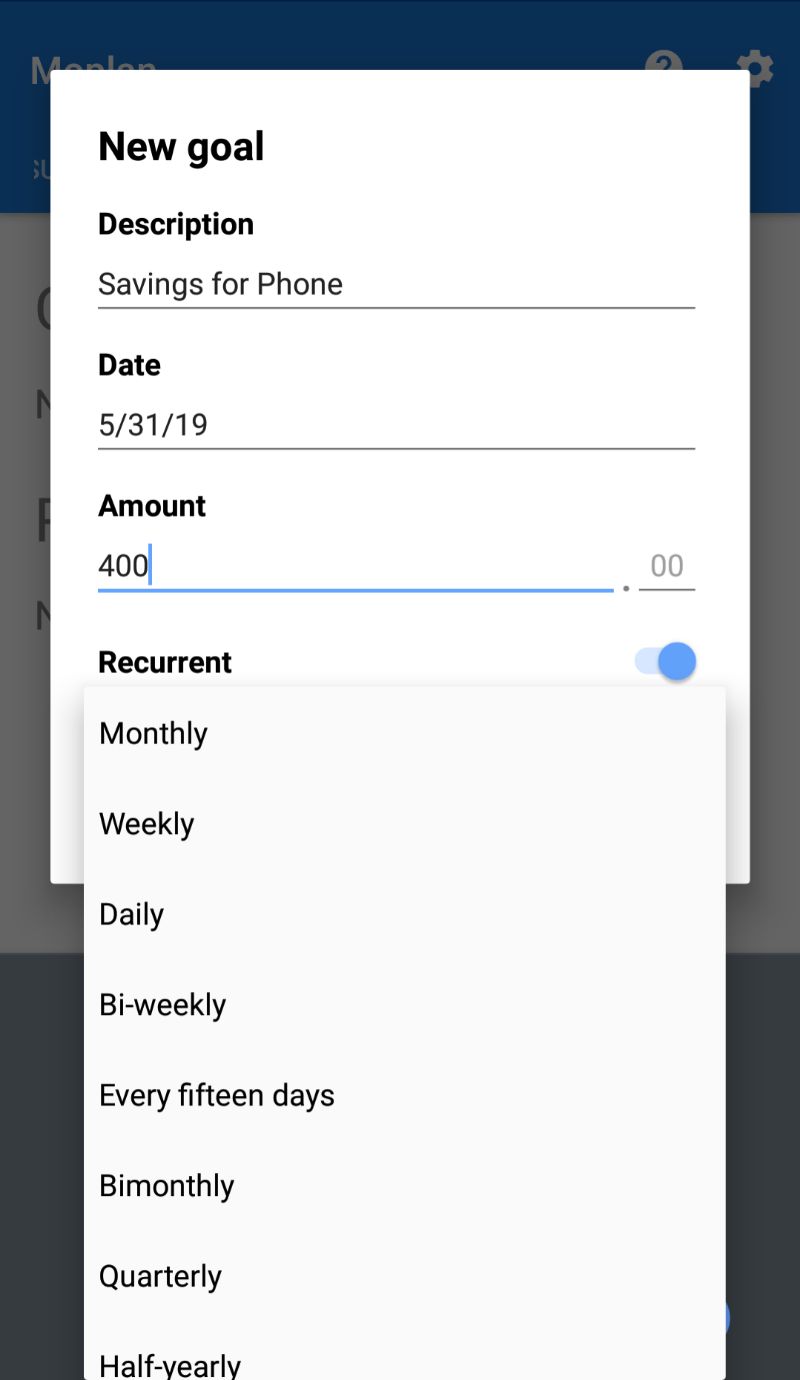This image is a screenshot of a budgeting app with a prominent pop-up window obstructing most of the background. The pop-up window, which is an opaque white box, is titled "New Goal." It contains four distinct fields laid out in a user-friendly format. 

1. **Description**: This field is filled in with the text "Savings for phone."
2. **Date**: The date section lists "5-31-19," formatting it as May 31st, 2019.
3. **Amount**: The amount field specifies a value of "400," with a blue cursor blinking after the zero, indicating that this line is currently active and underlined in blue.
4. **Recurrent**: This section is toggled on, meaning the savings goal is set to recur.

Below the recurrent toggle is an additional pop-up menu listing different recurrence options, such as monthly, weekly, daily, bi-weekly, every 15 days, bi-monthly, quarterly, and half-yearly.

The screenshot illustrates the budgeting app's interface, which is designed to help users set financial goals by entering a description, target date, desired savings amount, and specifying the frequency of deposits.